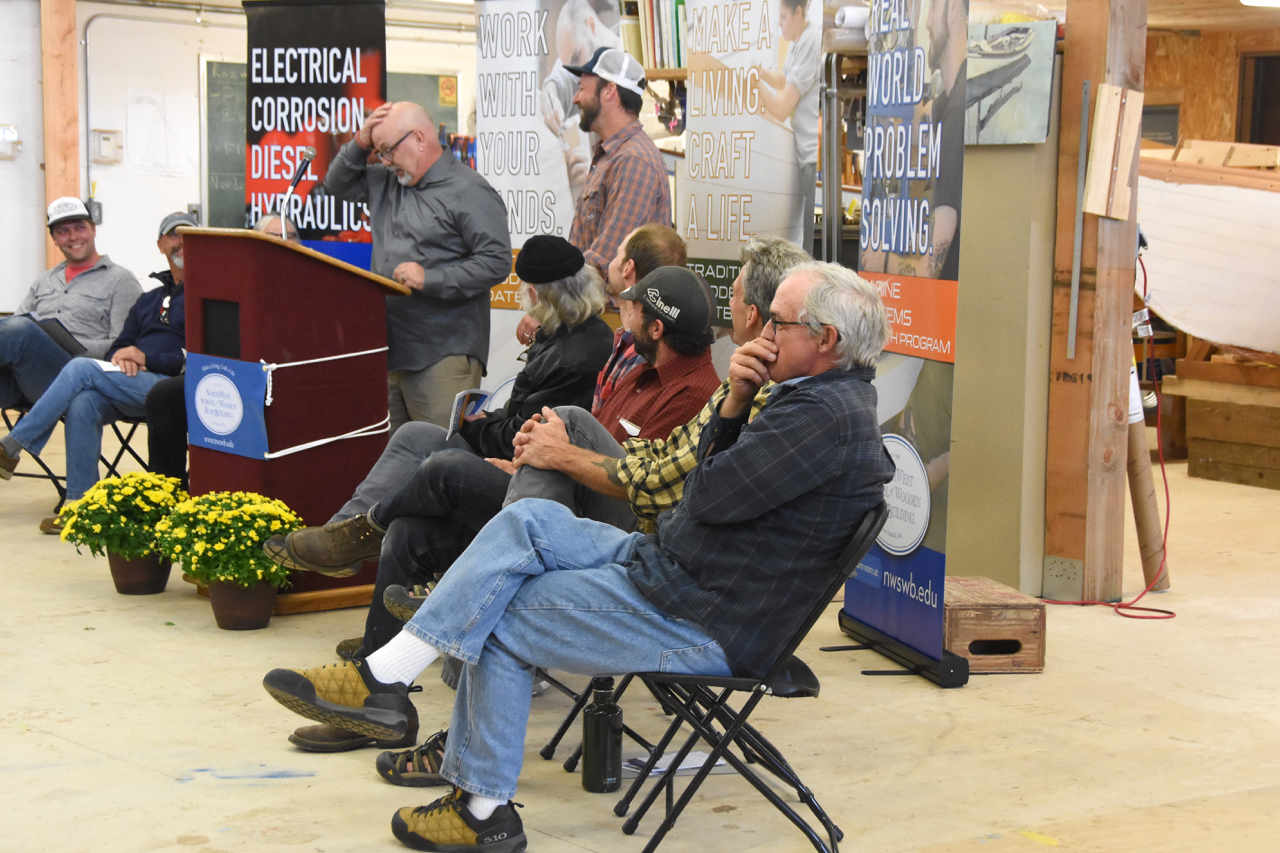The image is of an indoor work meeting or conference, potentially taking place in a woodworking shop. Central to the scene is a bald man with glasses standing at a brown podium adorned with a blue sign. He is wearing a long-sleeved gray shirt and has his right arm bent at the elbow, resting on the top of his head as he looks down, appearing contemplative. In front of the podium, there are two pots filled with vibrant yellow flowers. 

Seated in black folding chairs are seven men, some on either side of the podium. Five of the men are positioned to the left and appear engaged, with a mix of attentive and amused expressions - one man covers his mouth trying not to laugh. Behind the speaker, a man in a plaid shirt and baseball cap stands observing the scene. 

Decorating the backdrop are several banners with motivational phrases such as "Electrical Corrosion Diesel Hydraulics," "Work Better with Your Hands," "Make a Living, Craft a Life," and "Real World Problem Solving." The atmosphere suggests a professional yet informal setting, with individuals possibly in jeans or similar casual work clothing, all directed towards the speaker's presentation or talk.